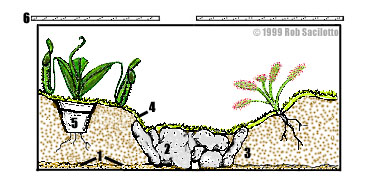This detailed digital illustration by Rob Sasioto, copyrighted in 1999, serves as an informative diagram for understanding plant growth, notably focusing on carnivorous plants. Set against a simple white background, the image displays an x-ray-like side view of the soil, revealing the roots and underground environment. On the left, there are three dark green plants, while the right features a plant with more yellow-green foliage and distinctive flowery, pinkish-white stalks, likely representing a carnivorous species. The soil beneath the plants is rendered with brown dots, and various elements are labeled with numbers from 1 to 6. For instance, stones are marked with number 2, and a pot with number 5, suggesting different components or stages of plant growth. Two bars at the top, possibly measurement tools, are marked with the number 6. The overall graphic, although simple and somewhat low in quality, effectively demonstrates the conditions needed for cultivating these unique plants, including the visual spread of roots and the interplay of soil and stones, aimed more at providing information than aesthetic pleasure.